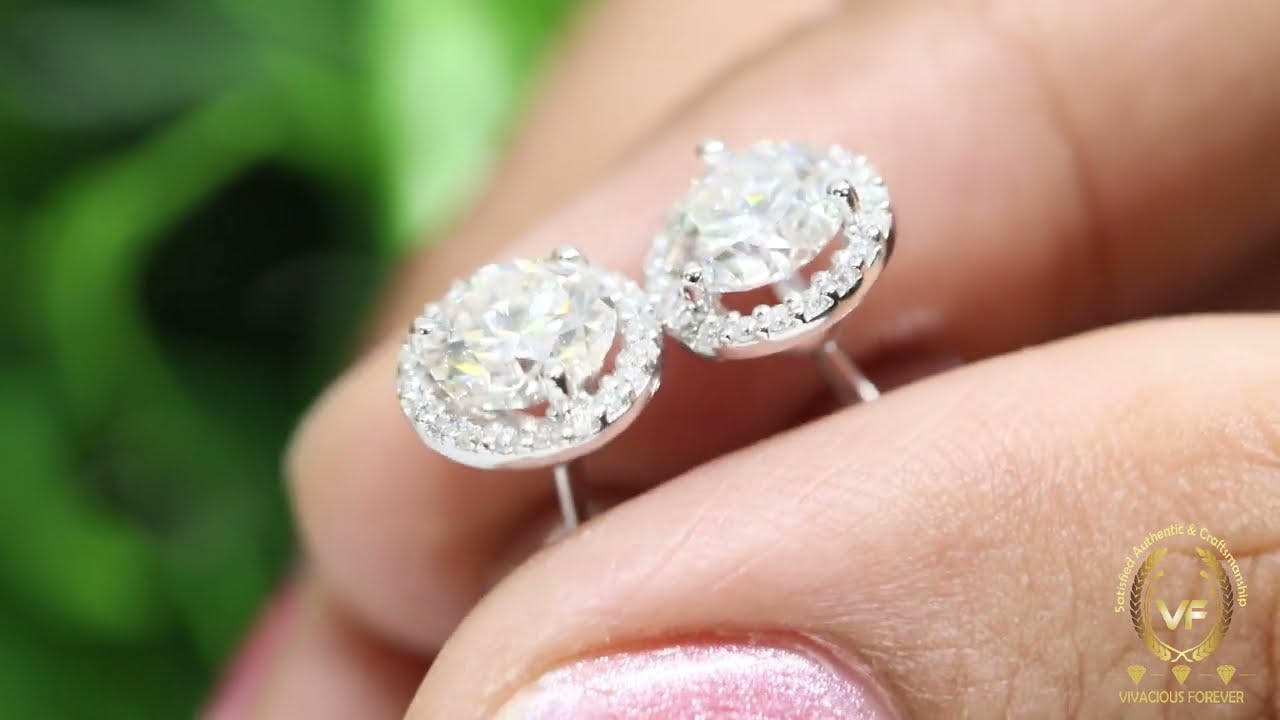In this professionally taken close-up photo, two intricately designed circular earrings are showcased. Each earring features a large central diamond encircled by a ring of smaller, glistening diamonds, all set in platinum or silver. The earrings are held delicately between the thumb and index finger of a woman’s hand, identified by her slender fingers and pink glitter nail polish. In the background, there is a blurred green element, possibly foliage, that adds a touch of nature to the setting. The overall color palette of the image includes green, gold, black, white, silver, peach, and pink. The bottom right corner of the image contains a gold emblem with the text “VF, Vivacious Forever," suggesting a high-end, detailed presentation suitable for a jewelry advertisement.